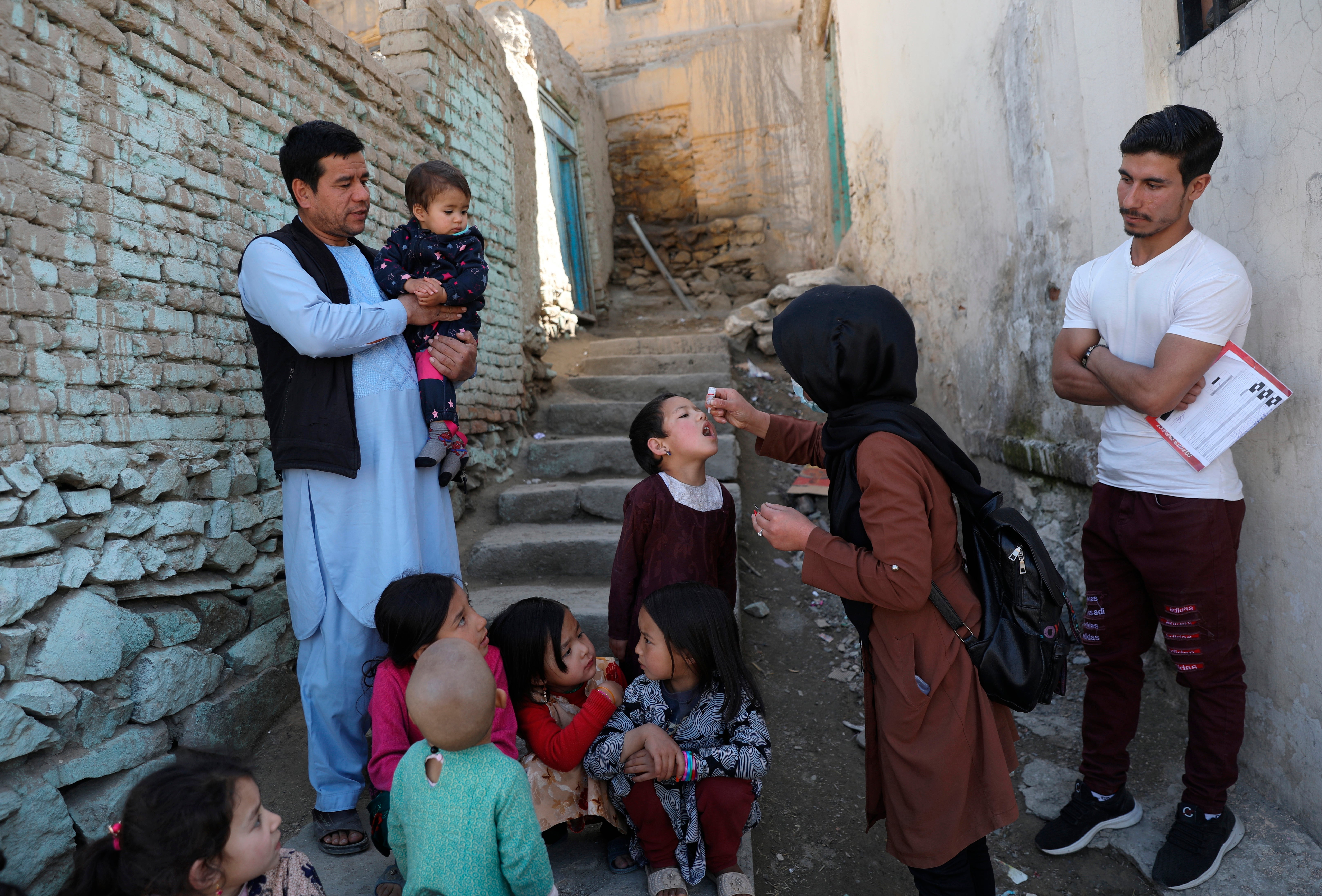This is a color photograph capturing a scene in an alleyway where medical workers are administering medicine to children. The narrow alleyway has stone steps ascending at the back, bordered by a tan-colored brick wall on the left side that has remnants of blue paint and a deteriorating white wall on the right side. On the left, a man dressed in a light blue shirt, blue pants, and a blue vest is holding a toddler. On the right, another man in red pants, black shoes, and a short-sleeve white shirt, is holding a piece of paper. Adjacent to him, a woman in a black headscarf, long-sleeved brown coat, and black pants is using a white droplet bottle to administer medicine to a standing child. Several other children are seated on the ground, likely waiting their turn for the treatment. The scene is indicative of a medical outreach effort in a Middle Eastern setting.